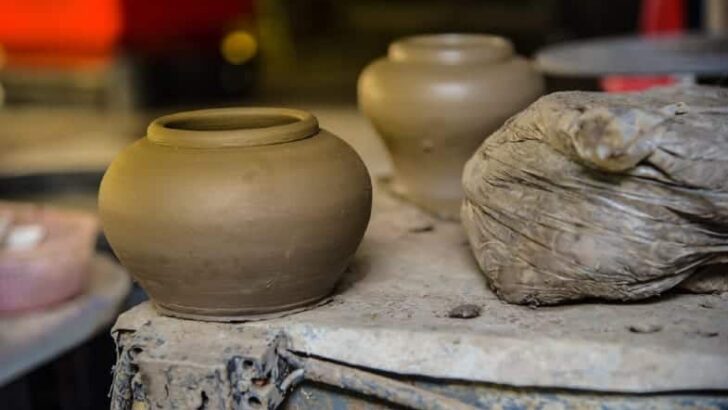This photograph captures the rustic ambiance of a potter's workshop, highlighting a central brown clay pot situated on the edge of a weathered, grayish-white surface that is rough and dusty. The pot, which has yet to be painted or fired, features a small rim, a large body, and a narrow base. Adjacent to it on the right stands a large grayish-white sack that resembles a bag of materials used in pottery. Blurred into the background are additional ceramic items including another brown pot, tables, and assorted objects with shades of pink, orange, and black. The workspace, replete with metal hinges and a mix of stone or cement surfaces, exudes a sense of active, creative disarray, typical of an artisan's studio.